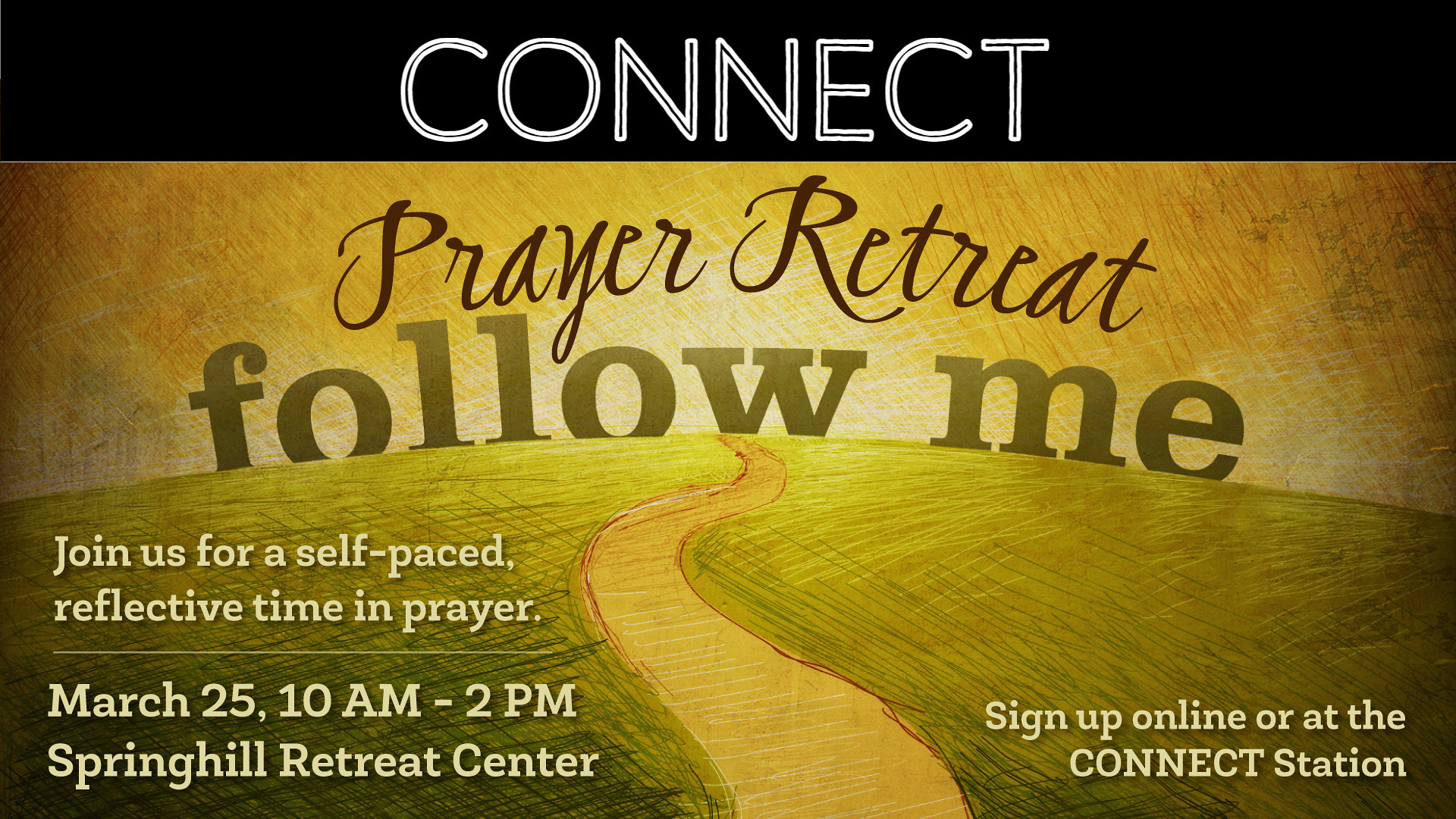The image is a detailed advertisement for a prayer retreat. At the top, a black banner with white text prominently reads "Connect," featuring a black line through the center of each letter. Below, a strip of yellow background evokes a sunrise, with the text "Prayer Retreat" in dramatic brown letters and "Follow Me" in grayish-yellow text. The image illustratively depicts a yellow walking path flanked by grass, symbolizing a journey towards the sun—an apt metaphor for the retreat. The lower portion provides essential details in greenish-yellow text: "Join us for a self-paced reflective time in prayer. March 25th, 10 a.m. to 2 p.m., Spring Hill Retreat Center. Sign up online or at a Connect station," with the date on the lower left and additional information on the lower right.